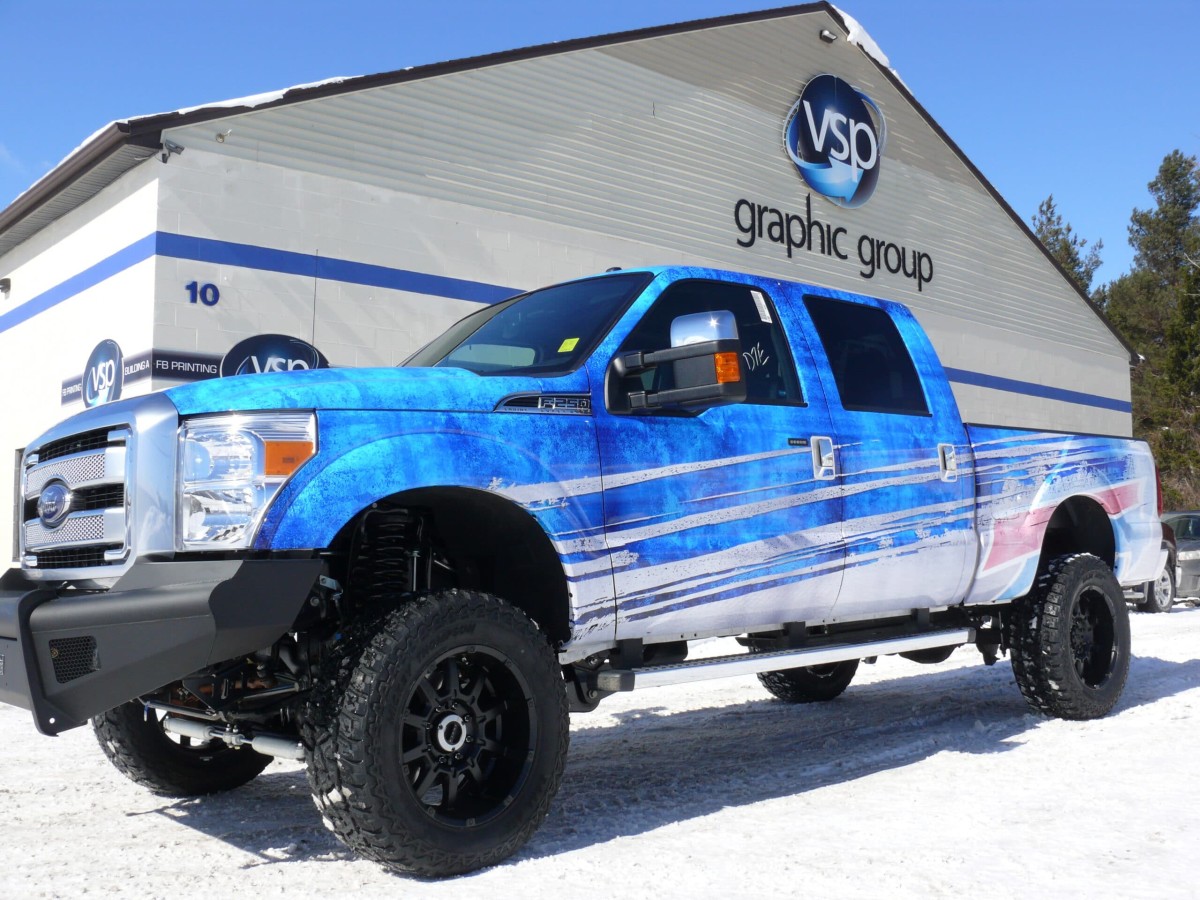The image is a detailed color photograph of an impressive and heavily customized Ford truck, likely an F-150, F-250, or F-350, with a double cab and large 4x4 build. The truck is adorned in an eye-catching wrap featuring varying shades of blue with marbling effects, along with long, white streaks that give the appearance of snow being thrown down its sides. There's also a subtle red stripe on the back. This snowy scene clearly places the truck outdoors in winter, with snow on the ground, wedged in the tire treads, and even dusting the roof corners. 

The truck is parked in a lot outside a white, warehouse-like building belonging to VSP Graphic Group, identified by a logo prominently displayed at the top middle of the building facade. Additionally, a blue stripe runs all around the side of the building, which is marked with the number 10 at the bottom left corner. The background features some trees and a glimpse of another vehicle's wheel at the bottom right, adding further context to this crisp winter setting. The bright blue sky peeks through, completing the vivid and dynamic scene as the truck stands as a testament to the high-quality graphic work presumably offered by the company.